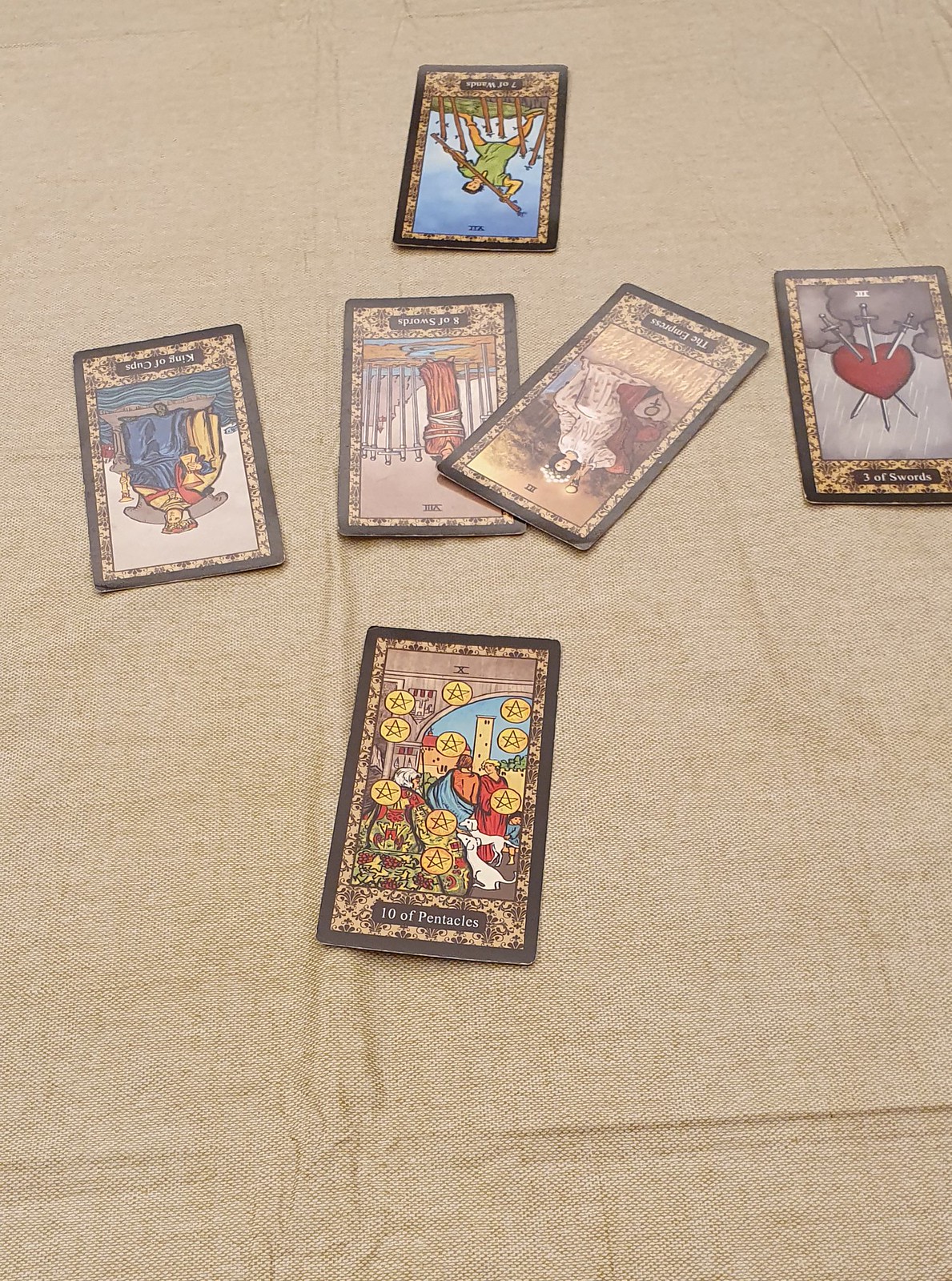The image depicts a series of six tarot cards arranged on a light brown tablecloth. The central card is the "Ten of Pentacles," which is face-up. This card is enclosed in brown and light brown borders adorned with floral designs. The central imagery features a blue sky background, with two old-fashioned figures dressed in capes and long gowns, standing amid castle-like buildings. White animals also appear in the scene. Golden stars, ten in total, with one dark star outlined in the middle, dot the card.

On the upper left, there are two cards placed upside-down. The first of these is the "King of Cups," featuring a person in a long blue gown and a beige cape, holding a cup and possibly a sword. The person appears to bear a crown, suggesting royalty. The background showcases water elements.

Next to it, also upside-down, is the "Eight of Swords." This card depicts a figure in a long red covering bound with white ropes, set against a brown sky with mountains in the backdrop. A fence is also visible in the scene.

To the right, at an angle and upside-down, is another card featuring a girl in a long white dress and a hat. She appears to hold a flashlight, against a beige sky with clouds. The text on this card is unreadable.

The fourth card, the "Three of Swords," is upright. It shows gray clouds and a red heart pierced by three swords, with their tips sticking out at the bottom. The card's title is inscribed in a black box at the bottom.

At the top, there is a card showing a man in a green outfit holding a stick or a sword. Several other sticks are planted in the ground in front of him. The background reveals some greenery. The text on this card is also unreadable due to the image quality or positioning.